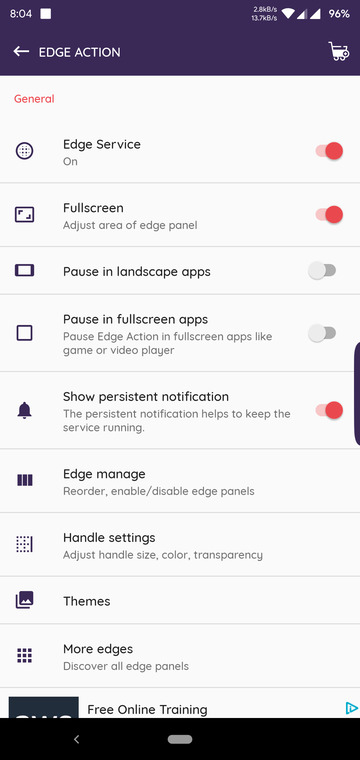The image appears to depict a smartphone screen captured in a vertical orientation. At the very top of the screen, to the left, the time is displayed as "8:04." Adjacent to the time is a small square box, followed by a black space. Continuing to the right, icons indicate the Wi-Fi signal and battery level, which reads as 96%. Further right, a small black space is visible, followed by a left-facing arrow labeled "Edge Action." Another black space is present on the far right, which contains an indistinct icon that resembles a shopping cart.

The main portion of the screen is set against a white background. The first item at the top is labeled "General" in red text, accompanied by an icon. Below this, it states "Edge Service" next to an active red toggle button.

Following this, there is an option for "Adjust area of landscape apps" with a corresponding icon; this toggle is set to the off position. The next section is labeled "Pause full screen apps," which includes a description that reads "Pause edge action in full screen apps like games or video player," with the toggle also set to off.

Further down, the screen lists several options:
- "Show persistent notification," with an icon beside it.
- "Edge manage," with an accompanying icon.
- "Handle settings," with an icon.
- "Themes," accompanied by an icon.
- "More edges," with an icon.

At the bottom, there is a section offering "Free online training," marked by a forward arrow and followed by another black bar.